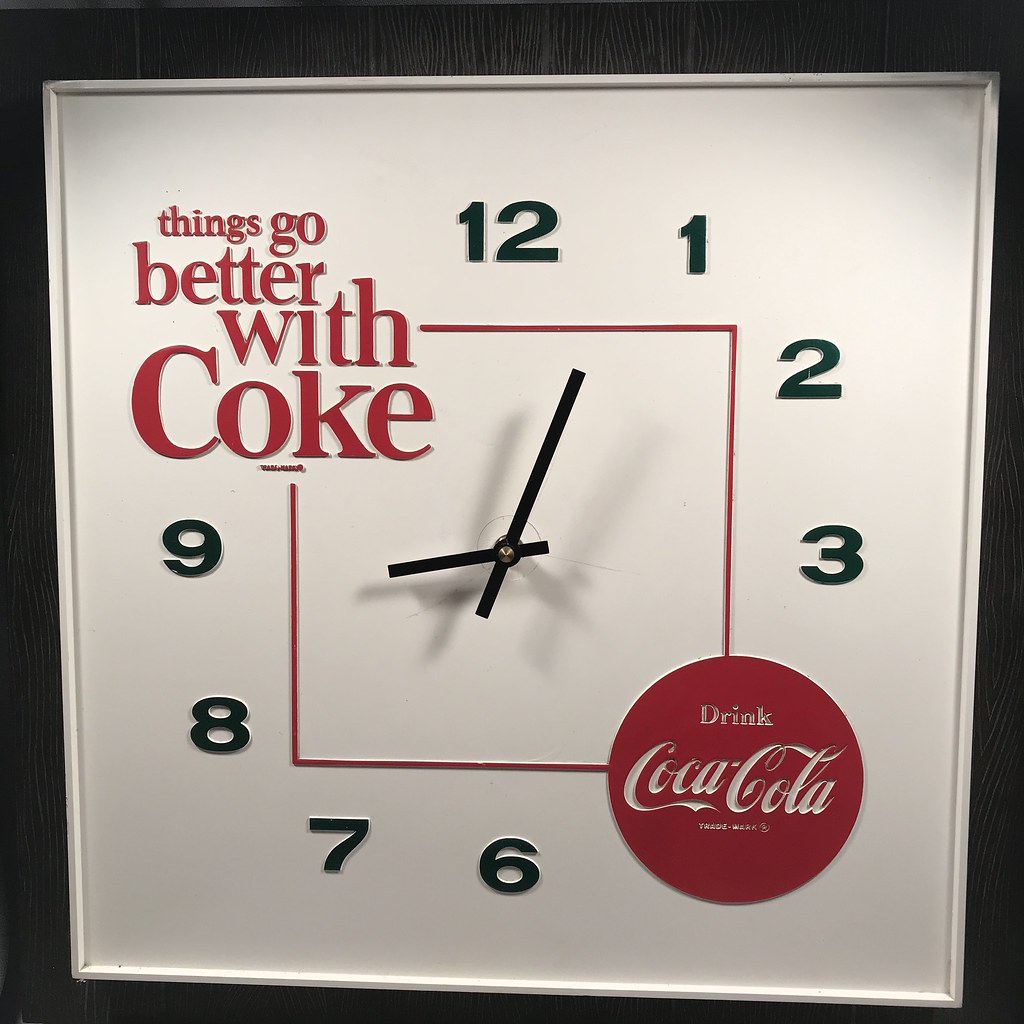This is a photograph of a Coca-Cola branded square analog wall clock, likely a promotional item intended for restaurants or grocery stores. The clock features a clean white face with a whitish frame and a silver border. Prominently displayed on the clock are various Coca-Cola advertisements. In the upper left corner, there is red text that reads "Things go better with Coke," possibly accompanied by a small, hard-to-see copyright notice.

The numbers on the clock are mostly typical black with white outlines, arranged in a circular pattern as on a traditional clock face: 12 at the top, followed clockwise by 1, 2, and 3, then resuming from 6 through 9. Notably, the 4 and 5 are replaced by a prominent red circular logo that says "Drink Coca-Cola" in white script. This logo disrupts the continuity of the numerical sequence but serves to reinforce the brand's presence.

Inside the numerical ring is an inner red square, adding a bold touch to the clock's design. At the clock's center, two black hands, one for the hours and one for the minutes, are secured with a gold fastening. The hour hand is positioned slightly after the 9, suggesting the time is approximately 9:03, although it seems slightly misaligned for perfect accuracy.

This clock merges function with brand promotion, adhering to Coca-Cola's classic red-and-white color scheme and iconic script to enhance its advertising impact.